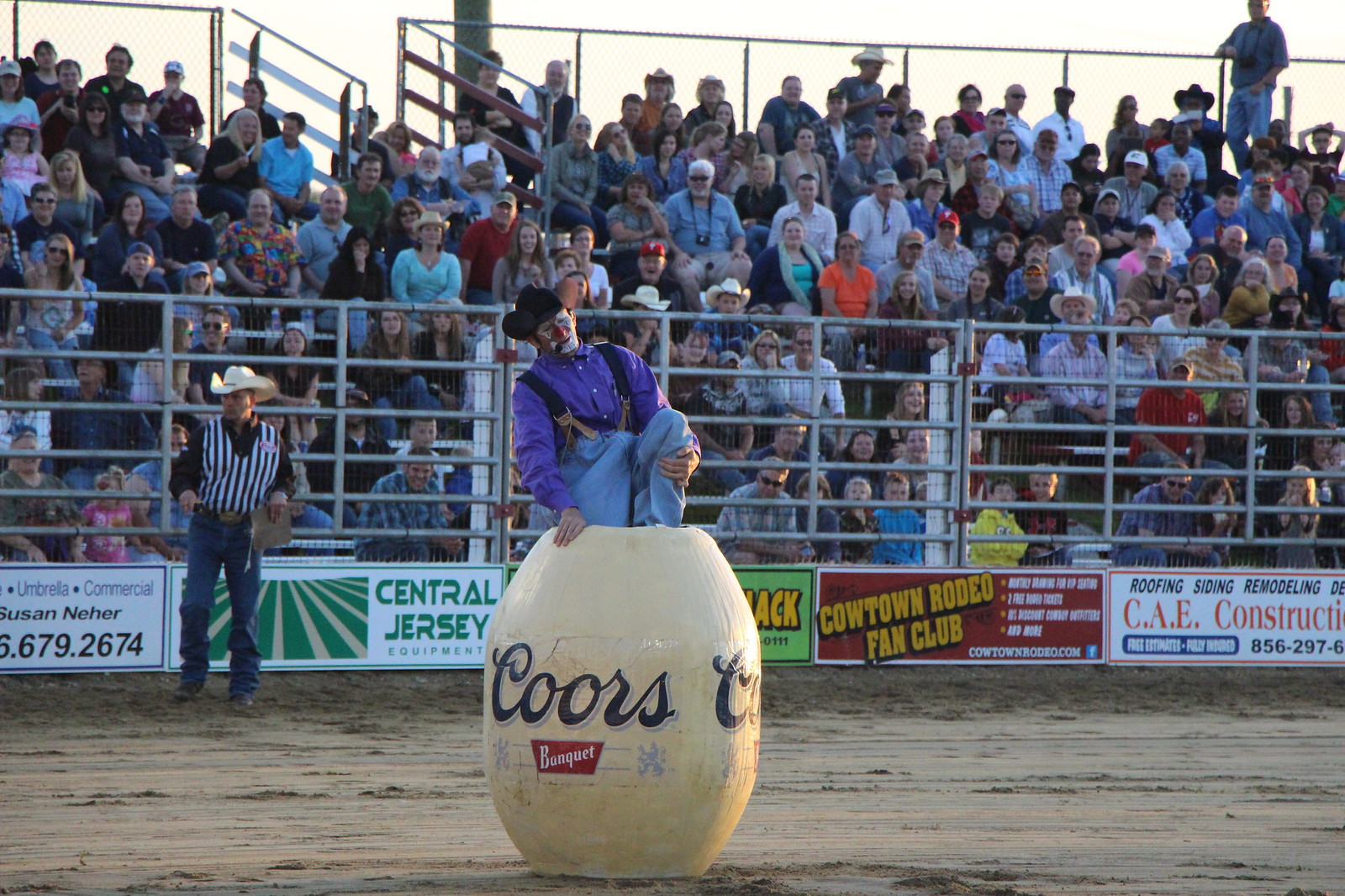The image captures a lively rodeo scene at dusk, featuring a rodeo clown and spectators. At the center of the sandy arena stands a rodeo clown dressed in clown makeup, a black cowboy hat, a purple shirt with a black vest, and signature blue baggy pants. He is seen climbing into a distinctive yellow, egg-shaped barrel that displays the Coors Banquet logo prominently, with "Coors" written in cursive and "BANQUET" in a small red trapezoid beneath it. Positioned behind the clown is a referee, identifiable by his white cowboy hat, striped referee shirt, blue jeans, brown cowboy boots, and a large belt buckle. The background showcases a bustling grandstand made of metal, filled with rows of spectators. Many are wearing cowboy hats, and some are standing, adding to the vibrant atmosphere of anticipation as they await the next event, likely the arrival of the bulls. The setting sun casts a warm glow over the entire scene, enhancing the anticipation and excitement of the rodeo.